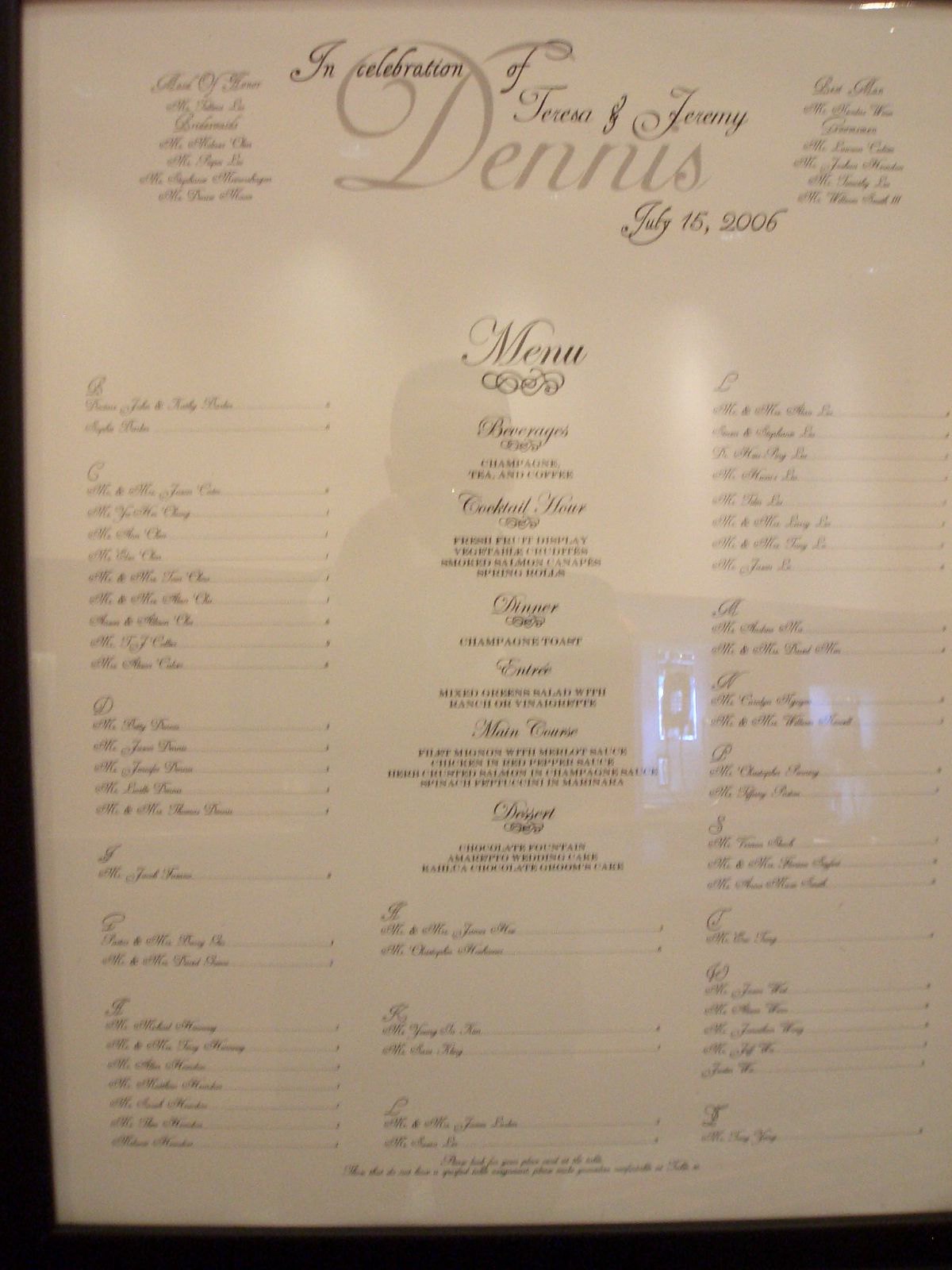The image features an elegantly designed wedding menu, printed on off-white paper with dark gray lettering. At the very top, in refined machine calligraphy, the text reads "In Celebration of Teresa and Jeremy," with the word "Dennis" prominently displayed in the background in large letters. Directly below this, the date "July 15, 2006" is inscribed.

The layout of the menu is divided into three main sections. On the left and right columns, there are lists of guests arranged by table, written in the same machine calligraphy style, though the text is too small to decipher. The central column, occupying the middle third of the image, features the detailed menu options, but these too are illegible due to their small size.

A notable detail in the image is the reflection of a man, presumably the photographer, captured on a shiny surface protecting the menu. The reflection shows the man standing in a well-lit room, holding a camera, with a wall and light source visible behind him.